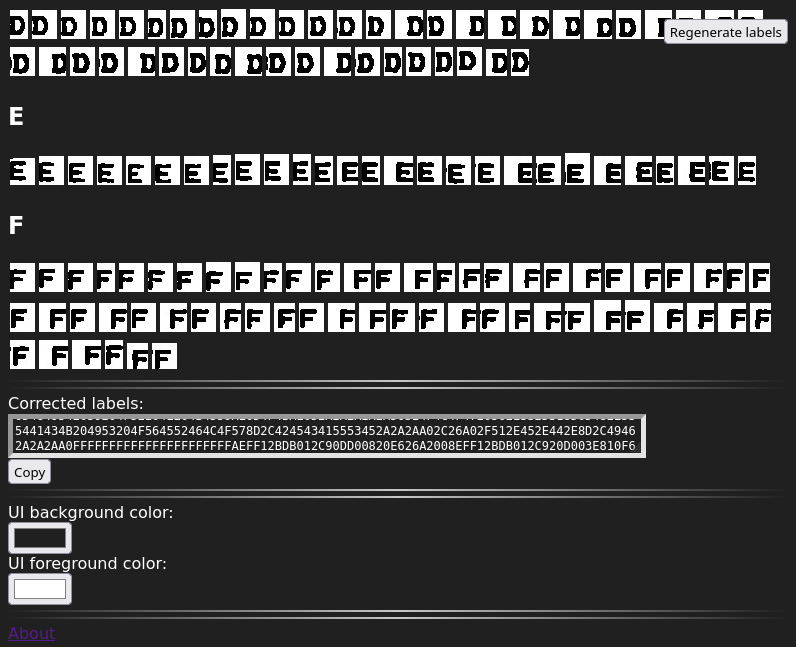This image depicts a large, dark gray interface box filled with various white sub-boxes, each containing different letters. At the top of the interface, there are two rows of white boxes: the first row contains over 20 boxes, while the second row holds about 15. Each box contains the letter "D," displayed in slightly pixelated fonts and varying alignments—some centered, others skewed to the left or right.

In the top right corner of the interface, a button labeled "Regenerate Labels" is visible. Below, there is a single row of white boxes displaying pixelated "E"s. Following this, the letter "F" appears along with three rows of boxes containing pixelated "F"s in diverse orientations, although the last row only features about six boxes.

There is a label reading "Corrected Labels" followed by a rectangular box filled with a lengthy string of code, containing numerous numbers and letters. Next to this code box is a button labeled "Copy." Additionally, the interface specifies "UI Background Color," with the indication of black inside the gray box, and "UI Foreground Color," marked as a whitish color within another grayish box. At the bottom, there is an "About" section written in purple.